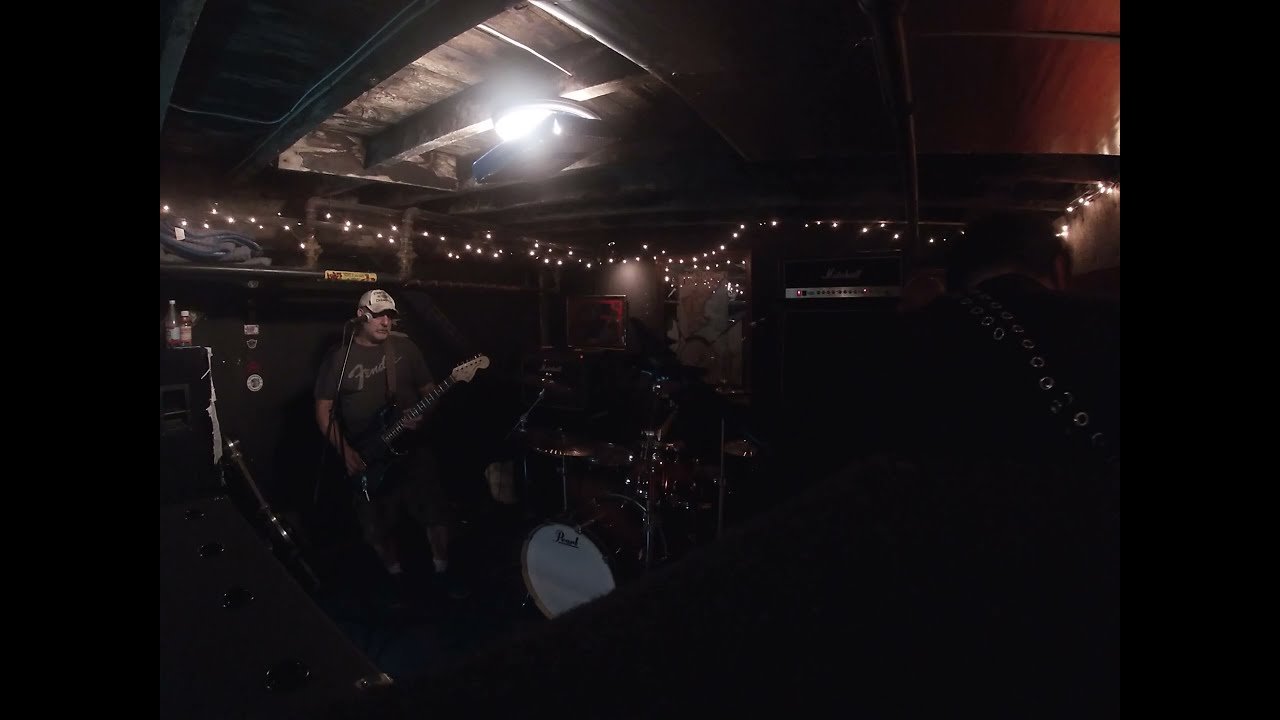In a dimly lit, possibly studio or bar setting, a man in a brown shirt and dark pants stands in the bottom left corner of the image, playing the guitar. He is illuminated enough to reveal his white baseball cap, worn forward, and his beard. Despite the darkness that envelops much of the scene, certain details stand out: dark brown wooden rafters stretch across a wooden ceiling on the top right, glowing string lights dangle behind the musician, and a bright white light hangs from the ceiling on the left side without focusing on anything specific. Scattered around are various equipment with blinking lights and drinks. A drum set is faintly visible in front of the guitarist, and to the right, another person with a guitar strap is turned away, adding a sense of depth to the space.